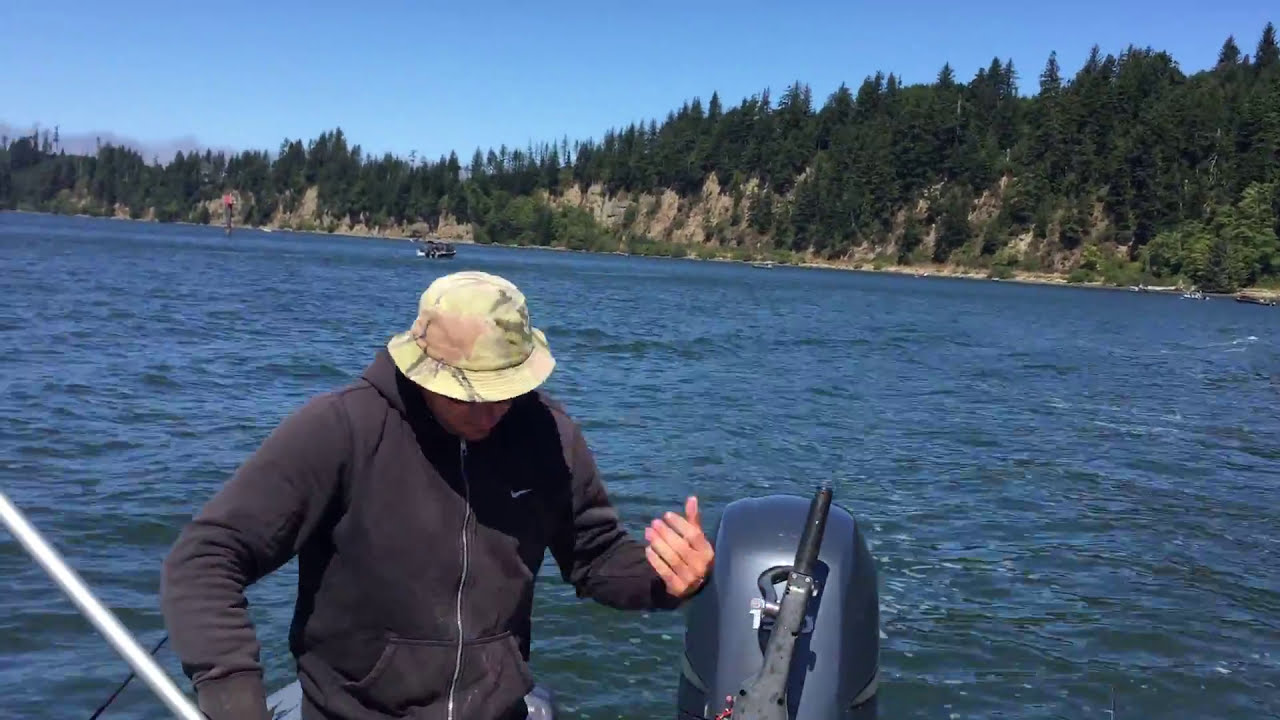This vibrant photo captures a sunny day on a lake, featuring a Caucasian man standing on a boat, partially seen from the waist up. He sports a brown fisherman's cap and a gray sweatshirt, zippered up, with his left hand visible but not his legs. His sweatshirt appears faded and may have a subtle Nike logo. His posture hints that he might be holding a pole or fishing equipment outside the frame.

The scene places the man near the boat's motor, centered at the bottom of the image. The backdrop showcases a brilliantly blue, gently rippling lake. Further in the background, a sloping hillside adorned with green trees and brown bluffs is visible under a bright blue, clear sky. The combination of blue water, green foliage, and brown landscape provides a striking contrast in the image, taken from the perspective of someone on the same boat, emphasizing the serene and picturesque outdoor setting.